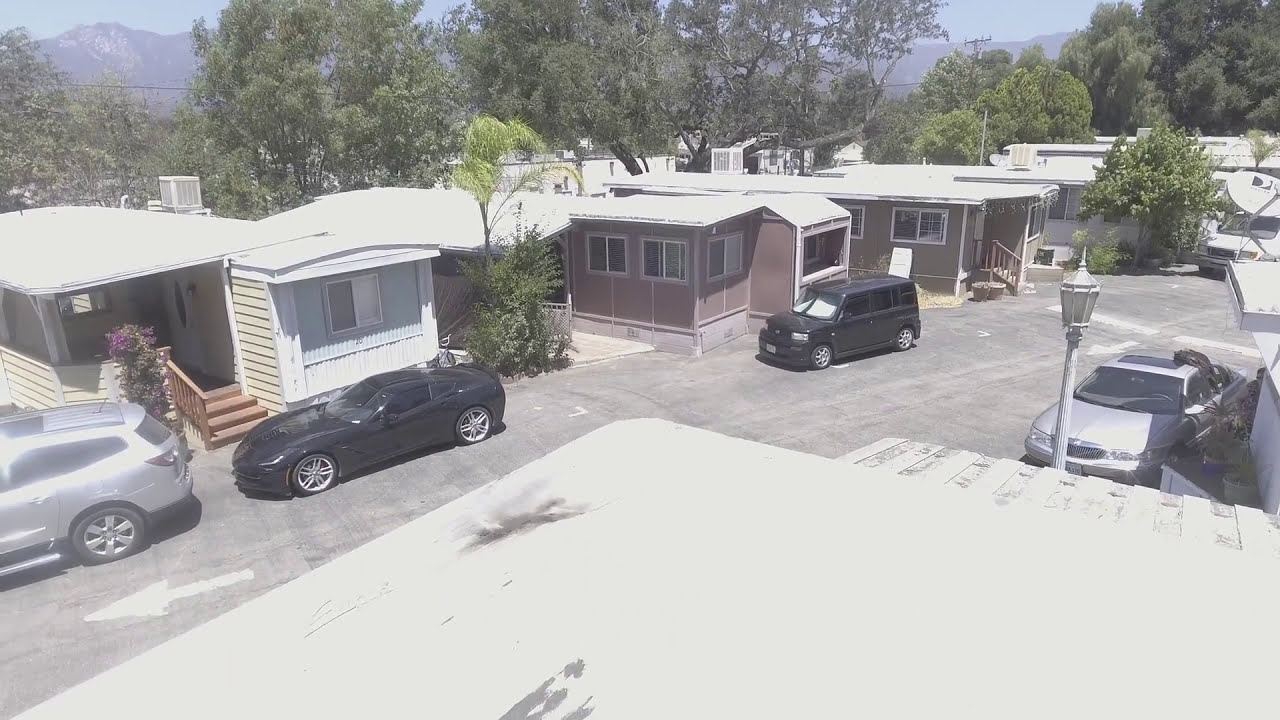This photograph, taken from a bird’s-eye view on a bright day, captures a small residential area, possibly a senior community. The gray one-way street runs diagonally from the middle right-hand side to the bottom left-hand side of the image, and it features some white markings. Parked along the street are four cars—two silver and two black. Lining the street are small, prefabricated houses with different colored sidings: a white-roofed house with green siding on the far left, followed by another with brown siding and a white roof, and lastly, a house with gray siding and a white roof. The bright sunlight makes the roofs almost blinding. Behind these homes, bright green trees are visible, and further in the distance, a tall, rocky mountain range partially obscures the blue sky. In the foreground, near the bottom edge of the image, a white roof-like structure suggests that the photograph was taken from an elevated position atop it.